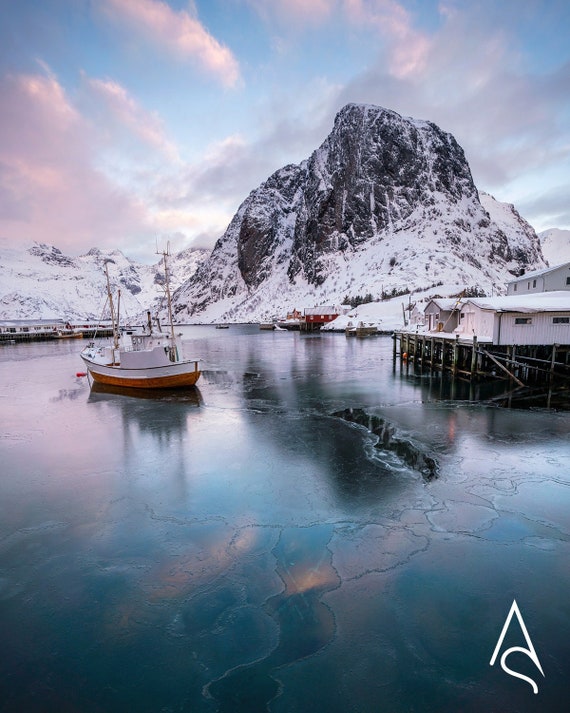The image captures a small fishing boat with a red bottom and white trim, floating on a lightly frozen lake in a serene, possibly Arctic or Alaskan, setting. The water reflects a mesmerizing sky filled with pink and blue hues, creating a beautiful sheen. To the right, a dock supports small houses extending over the water. In the backdrop, rugged snow-covered mountains tower under a sky adorned with pink-tinted clouds. The photo, which appears to be professionally taken and possibly in black and white, bears an artist’s signature resembling a squiggly 'A' in the lower right corner.